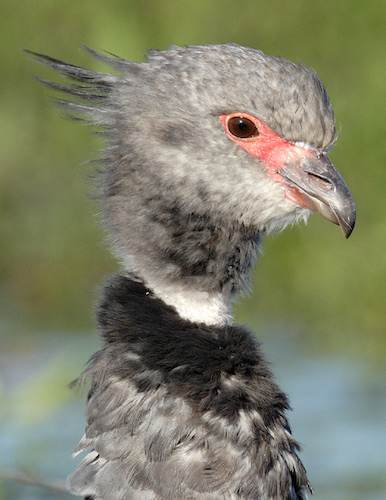This detailed and well-lit color photograph captures a close-up of a bird, possibly a young or old secretary bird, showcasing distinct plumage and features. The bird is viewed from the head to halfway down its chest, emphasizing its elongated neck and diverse feather colors and textures. Its head and neck feathers are predominantly grey with a small white patch at the base of the neck and a darker patch just below it. The area around its eye and the base of its beak is bare, exhibiting red, unfeathered skin similar to that of vultures or chickens. The bird has a hooked grey beak, a large nostril, and brown eyes, possibly highlighted by a prominent brow. Feathers stick out like a crest from the back of its head.

The background is a blurred mix of green vegetation and possibly blue, suggesting water, creating an outdoor setting with bright lighting that may slightly fade the bird's colors. The bird's coat exhibits grey shades with variances, while the neckline presents a combination of black, grey, and a bit of white. The photograph is in portrait orientation, focusing sharply on the bird's head and neck, leaving the background and lower parts out of focus and indistinct.